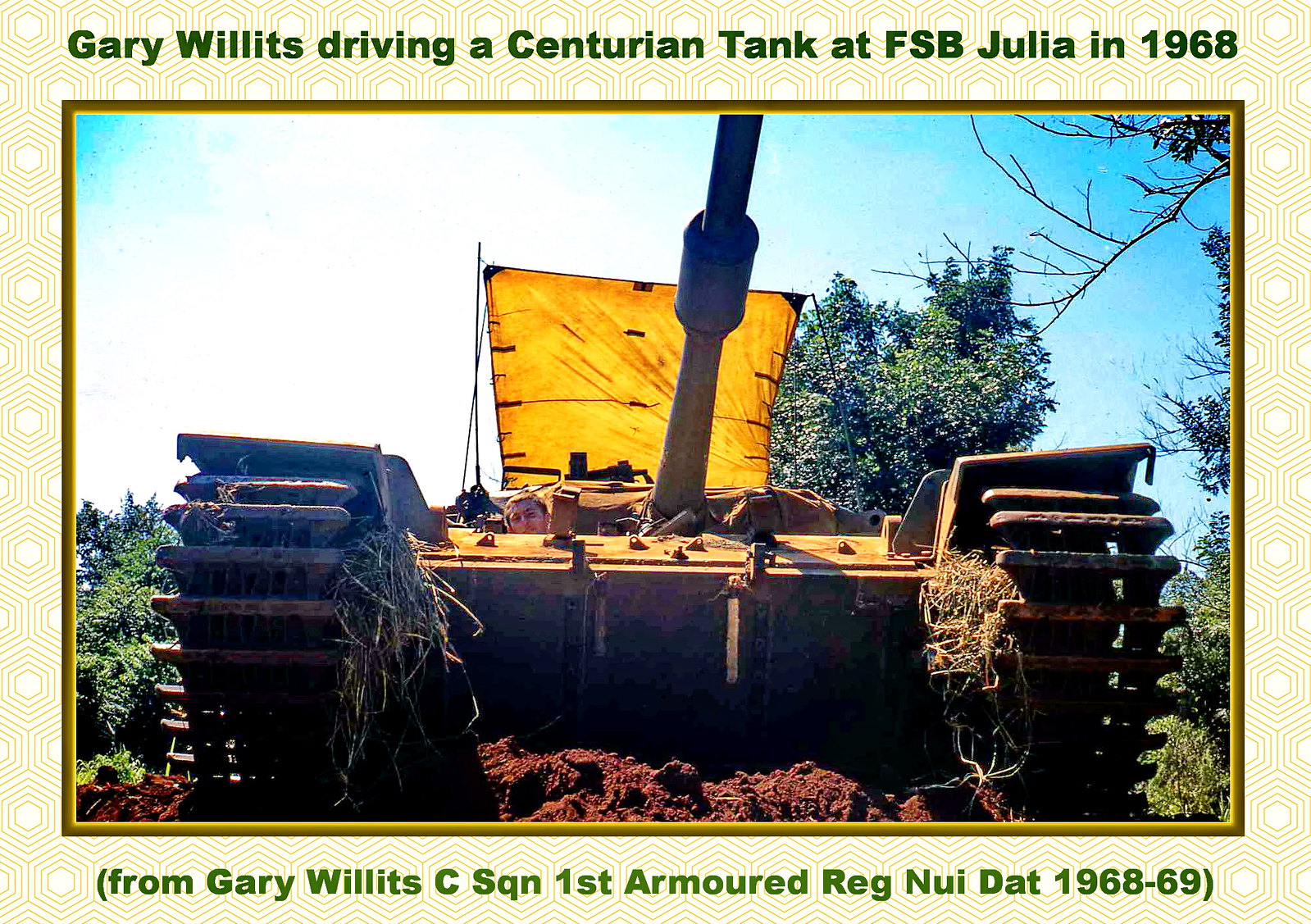The image captures a weathered Centurion tank, partially embedded in dirt and overgrown with hay or dried grass stuck in its tracks. At the top of the tank, a yellow tent-like shade has been erected, under which a person’s head is visible, peeking over the top. The tank’s long barrel extends off the frame, pointing outward. The photo, taken from a downward angle looking up, also showcases a backdrop of trees, grass, and a blue sky. Text on the image reads: "Gary Willits driving a Centurion tank at FSB Julia in 1968" at the top, and "From Gary Willits, C-Squadron, 1st Armored Reg, Nui Dat, 1968-69" at the bottom.